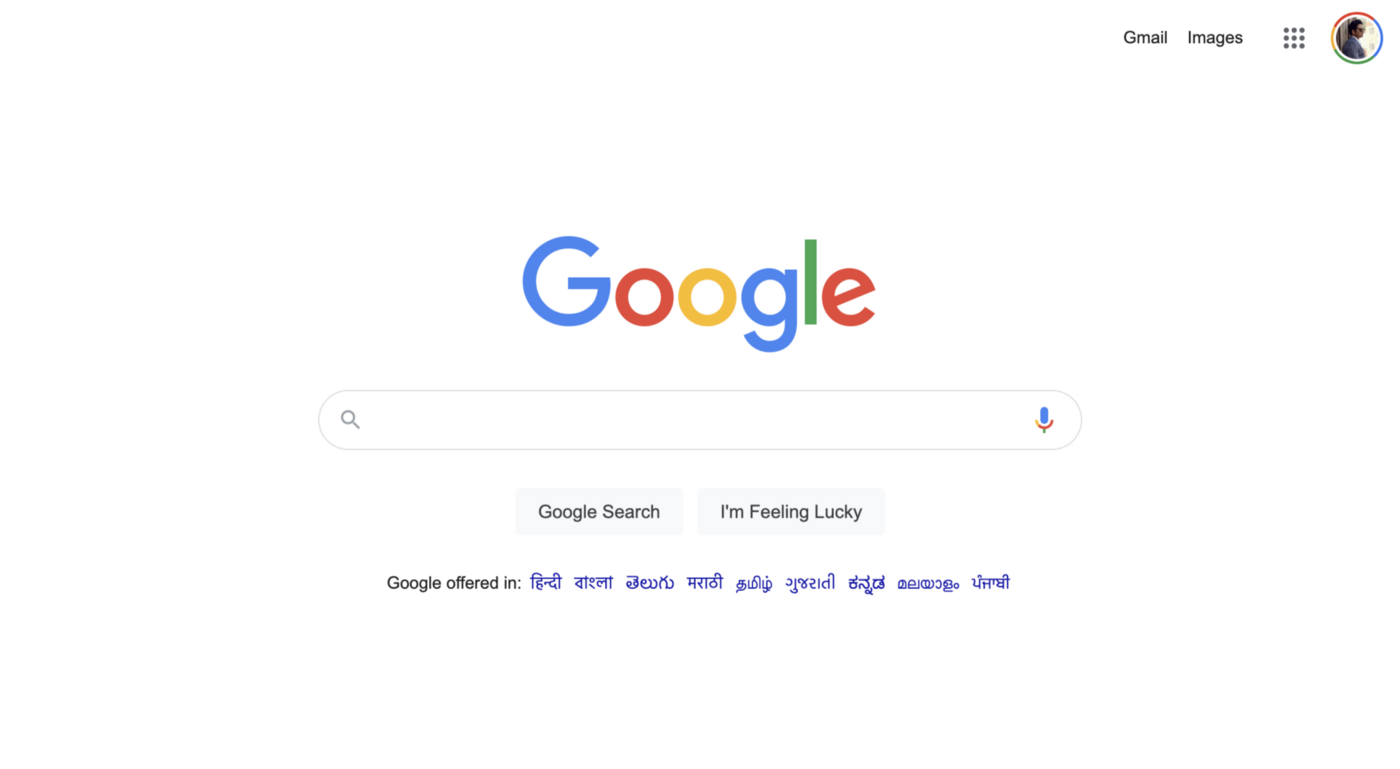The image depicts the Google search engine homepage on a standard desktop site, characterized by a clean, white background. In the upper right-hand corner, the words "Gmail" and "Images" appear in gray, followed by the Google Apps icon consisting of nine tiny dots. Next to it, the user's profile photo is visible, though it's extremely small and challenging to discern. It appears to be a side profile of a woman, possibly with a ponytail.

At the center of the page, the vibrant Google logo is displayed, showcasing its familiar blue "G," red "O," yellow "O," blue "G," green "L," and red "E." Directly below the logo is the search box, outlined in gray with rounded corners. On the left side of the search box is a magnifying glass icon, while on the right side is a microphone icon, indicating that voice search is available.

Underneath the search bar, two buttons are visible: "Google Search" on the left and "I'm Feeling Lucky" on the right. At the bottom, there's a line of text stating "Google offered in," followed by non-Latin characters that seem to represent a foreign language, though it's not immediately clear which language it is.